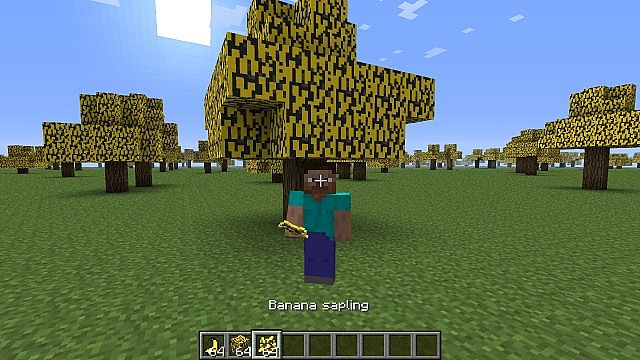A vibrant Minecraft scene captures the essence of the popular game with its distinct blocky aesthetic. The sky is a clear blue, contrasting with the lush green ground below. Prominently displayed at the bottom are nine inventory slots. The first three slots each hold 64 units, represented by icons resembling a banana, a cube, and possibly an owl.

Above the inventory slots, white lettering spells out "banana sapling." Dominating the central area of the screenshot is a character avatar clad in a blue t-shirt and dark navy-blue pants, seemingly holding a banana. The avatar's head appears brown, adding ambiguity to whether they are facing towards or away from the viewer.

In the backdrop, a large square-shaped tree towers directly above the character, anchoring the scene. Spanning the horizon, numerous similar trees stretch outwards in pairs, gradually diminishing in size with distance. While the immediate foreground is devoid of flora, the horizon bustles with smaller, vividly green trees, enhancing the image's depth and visual intrigue.